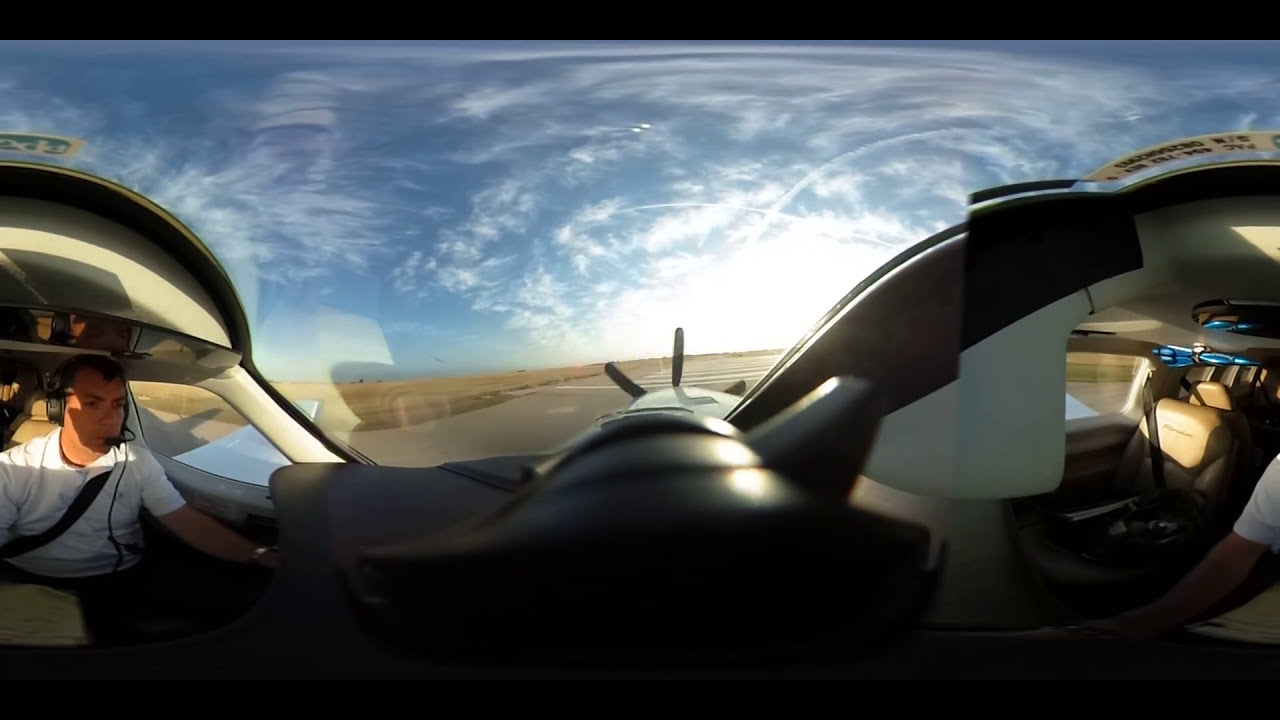The panoramic 360-degree image captures the interior of a light propeller aircraft, showcasing both the cockpit and the cabin. The viewpoint faces forward through the aircraft's windshield, revealing a bright blue sky adorned with thin, wispy clouds and a sun low on the horizon. Outside, a runway with white markings extends into the distance, flanked by a large field on the left.

The cockpit area on the left side features the pilot, comfortably strapped into his seat with a diagonal black seatbelt across his torso. Dressed in a white collared shirt and black pants, he wears a black headset with a microphone positioned near his mouth. A cable runs down the front of his body, likely connected to the headset. The pilot's left arm is extended along the length of the door panel, with his other arm resting near his seat. The aircraft's interior sports a neutral palette of light brown, off-white, or cream colors.

The front view through the windshield highlights the aircraft's three black propeller blades spinning at the front. To the right side of the image, there's an empty light brown leather seat equipped with a seatbelt. Several windows line the aircraft's sides, allowing sunlight to pour in and cast shadows within the cabin, emphasizing the brightness of the day.